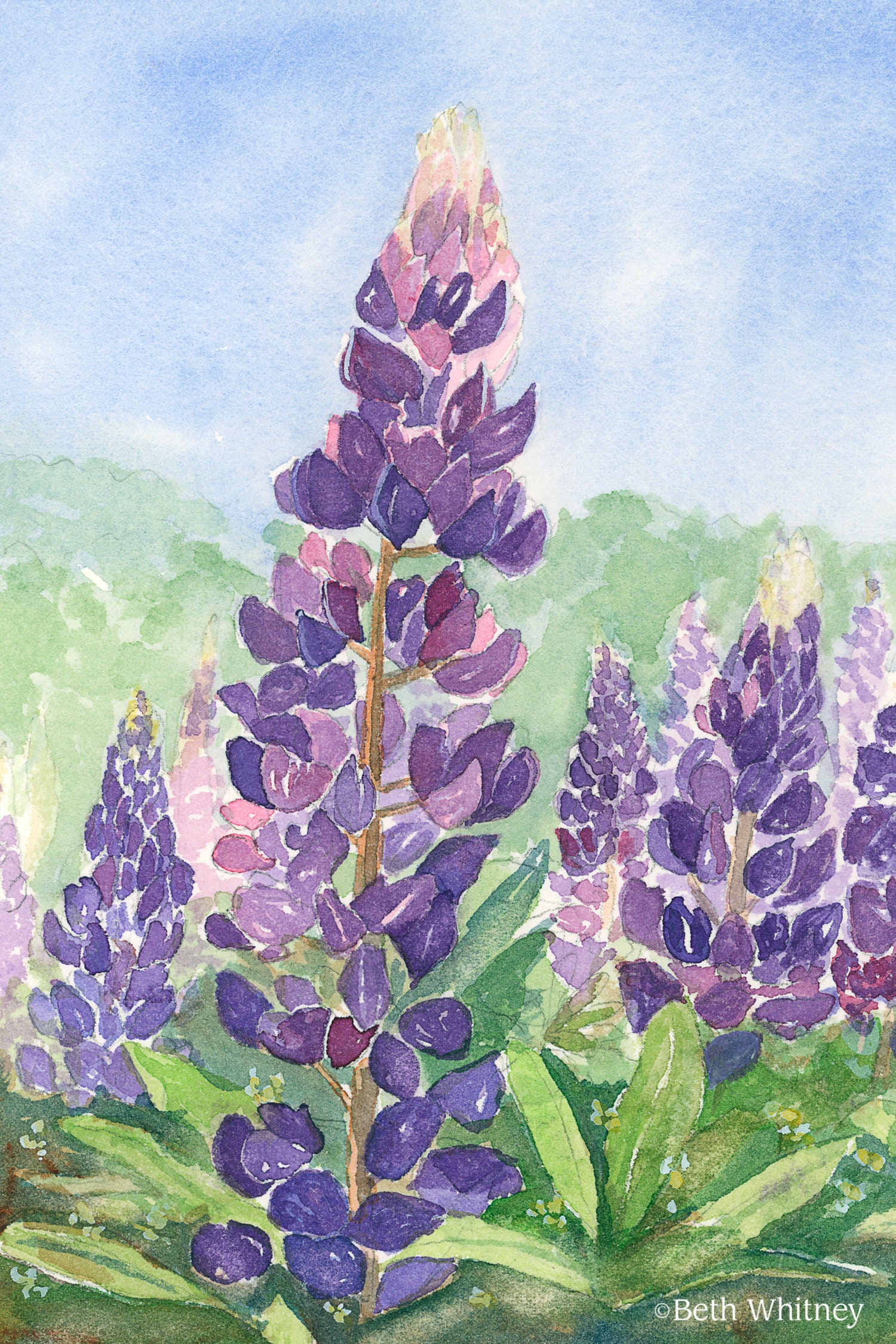This watercolor painting by Beth Whitney, with her name inscribed on the bottom right, illustrates a serene scene of purple wildflowers under a light blue sky with wispy clouds. The focal point is a tall flower stalk in the center, covered with dark and light purple buds, some tinged with pink and white. Surrounding this main flower are clusters of smaller, similarly hued blooms, interspersed with a few green leaves and even a solitary pink bud to the left. The background gradient transitions from a pale sky to a subtle green, suggesting blurred tree tops, adding to the depth and tranquility of the composition.